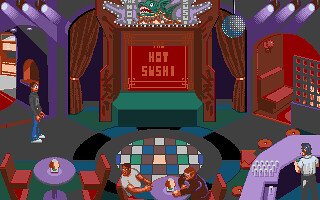The image depicts a pixel art scene reminiscent of 1980s video game graphics, showcasing a restaurant or bar titled "Hot Sushi." Dominating the center of the dining area is a stage with brown curtains, flanked by three spotlights on each side, and a disco ball hanging to the right. Above the stage, a sign reads "Hot Sushi." The establishment features purple round tables and reddish-brown chairs, with two patrons seated at one of the tables. To the bottom right, a purple bar hosts another person either polishing glasses or pouring drinks, and several glasses can be seen on the countertop. Adjacent to the bar, there's an additional seating arrangement that includes large couches. A solitary figure stands near the open space on the left side of the room. The color palette includes dark blue, green, yellow, and black, enhancing the nostalgic feel of the pixelated scene.